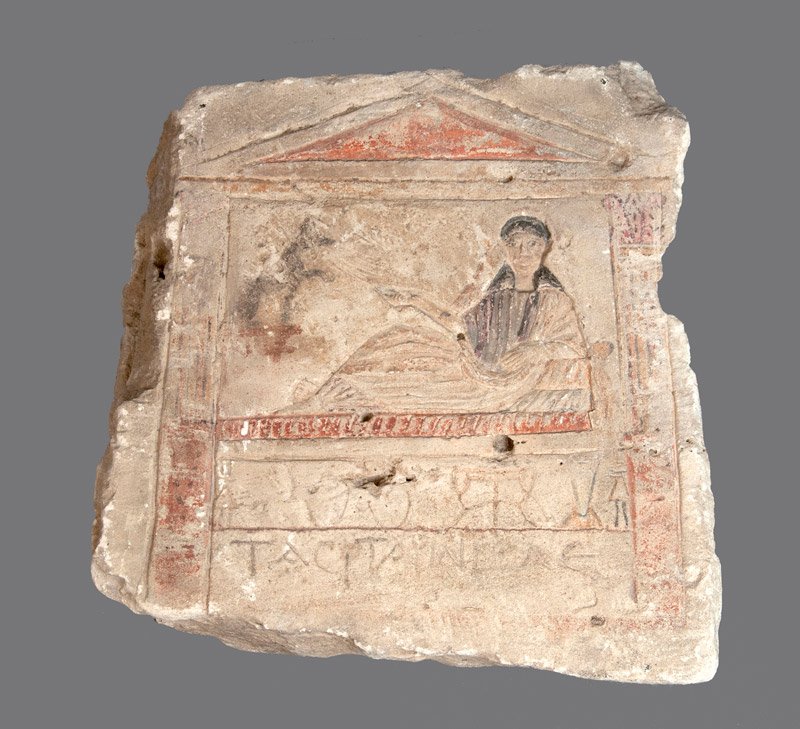The image depicts a highly weathered and ancient stone tablet against a dark gray background, showing signs of wear with frayed, broken edges. Etched into the whitish stone is a detailed scene featuring a woman reclining on what resembles a chaise lounge, partially propped up by a pillow or similar support under her elbow. The woman, possibly adorned in a flowing dress with a black shawl or headgear extending behind her neck and down to her shoulders, extends one hand outward toward an indistinct, weathered figure that might be an animal. Above her, an architectural feature, likely a Greek or Roman-style roof with red and orange trim, is held up by columns on either side. Beneath the etched figure is ancient, unreadable text, adding to the tablet's unique and historic aura. The entire scene is set on a dirt-covered surface, further emphasizing its age and antiquity.